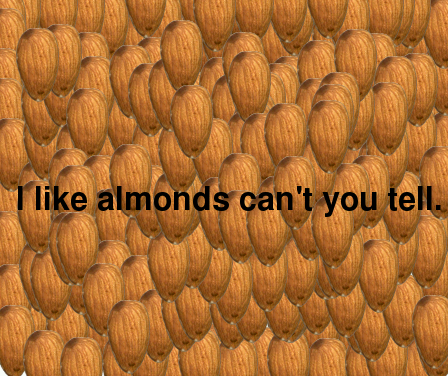This social media post features a visually striking, artistic image dominated by an irregular, overlapping pattern of dark brown almonds, each with a thin, pointed end facing downward and topped with a very dark brown spot. The entire background is saturated with these almonds, creating a dense, scale-like texture with virtually no space between them. In the foreground, centered almost exactly in the middle of the image, a bold black text statement reads, "I like almonds, can't you tell?" The juxtaposition of the text against the almond backdrop underscores the evident passion for almonds, emphasizing the playful and somewhat humorous nature of the post.